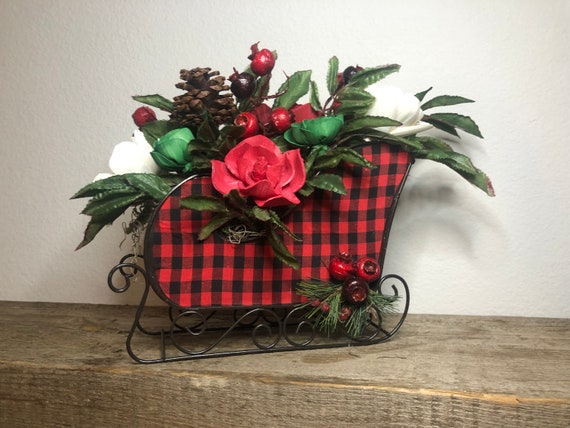This photograph showcases a festive Christmas sleigh ornament perched on a wooden slab. The sleigh is adorned in a striking red and black buffalo check pattern with thin black metal treads featuring delicate curls. Inside the sleigh, a charming arrangement of holiday elements provides a vibrant splash of color against the white wall background. The floral ensemble includes a mix of red roses, white flowers, and pine cones, interspersed with lush green leaves. Accentuating the festive spirit, there are red berries and small pomegranates or cherries placed within and glued to the sides of the sleigh. At the bottom back, a sprig of mistletoe delicately dangles, adding a traditional Christmas touch. The sleigh faces to the left, creating an elegant display that captures the cheer of the holiday season.